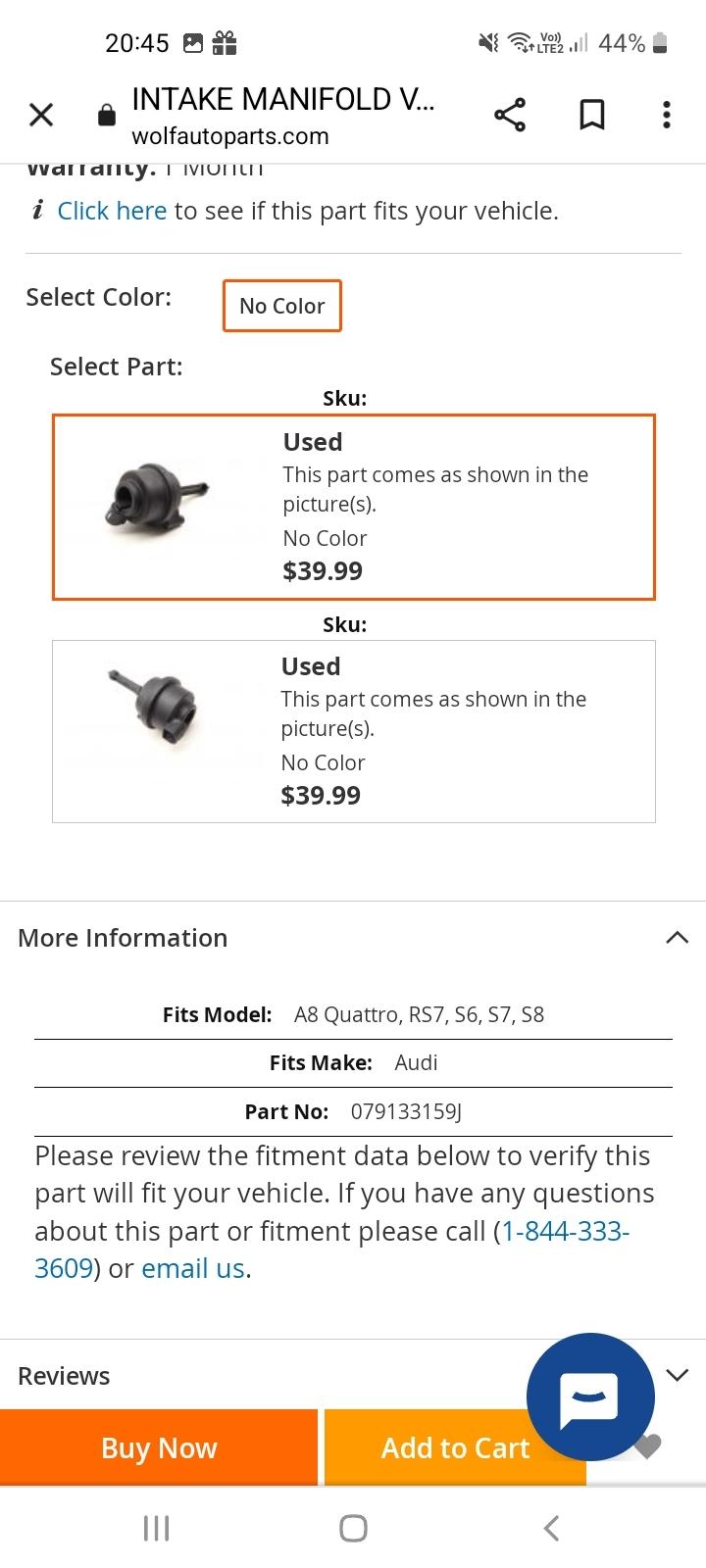**Screenshot of WolfAutoParts.com Browsing Experience on Android Device**

The screenshot showcases the user interface of an Android device with the website WolfAutoParts.com open. In the lower-left corner, the classic Android navigation icons are visible: the three vertical lines for recent apps, the square for home, and the triangle for back.

The device's status indicators indicate it is 8:45 PM. The phone is silenced, Wi-Fi connectivity is at full strength, and the LTE signal is at half strength, displaying two out of four bars. The battery is at 44%.

The webpage displays an item listing for an intake manifold with a truncated label "intake manifold V...". The webpage is from Wolf Auto Parts (wolfautoparts.com) and is primarily intended for vehicle parts shopping.

Visible elements include:
- An image icon and a gift icon, suggesting multimedia content and promotional offers.
- Functional icons such as an 'X' to close, a padlock for secure browsing, a share icon, a bookmark icon, and three vertical dots for additional options.
- A warranty notice stating "one month warranty."
- A clickable information link prompting, "Click here to see if this part fits your vehicle."

The product description provides detailed information:
- The intake manifold has no color selection and is priced at $39.99.
- It is described as "This part comes as shown in the pictures" with emphasis on its no-color designation, highlighted in orange.

The compatible vehicle models are listed as:
- Audi A8 Quattro, RS7, S6, S7, and S8.
- The part's designated fit make is Audi, with the part number 079133159J.

Additional information requests users to verify the compatibility of the part with their vehicle using fitment data. Customers are encouraged to contact customer service at 1-844-333-3609 or via email for further inquiries. Both contact options are clickable links.

User interaction elements like "Buy Now" and "Add to Cart" buttons are prominent, alongside a pop-up chat option for immediate assistance.

The screenshot effectively shows a user browsing and considering purchasing an automotive part on WolfAutoParts.com from an Android device.